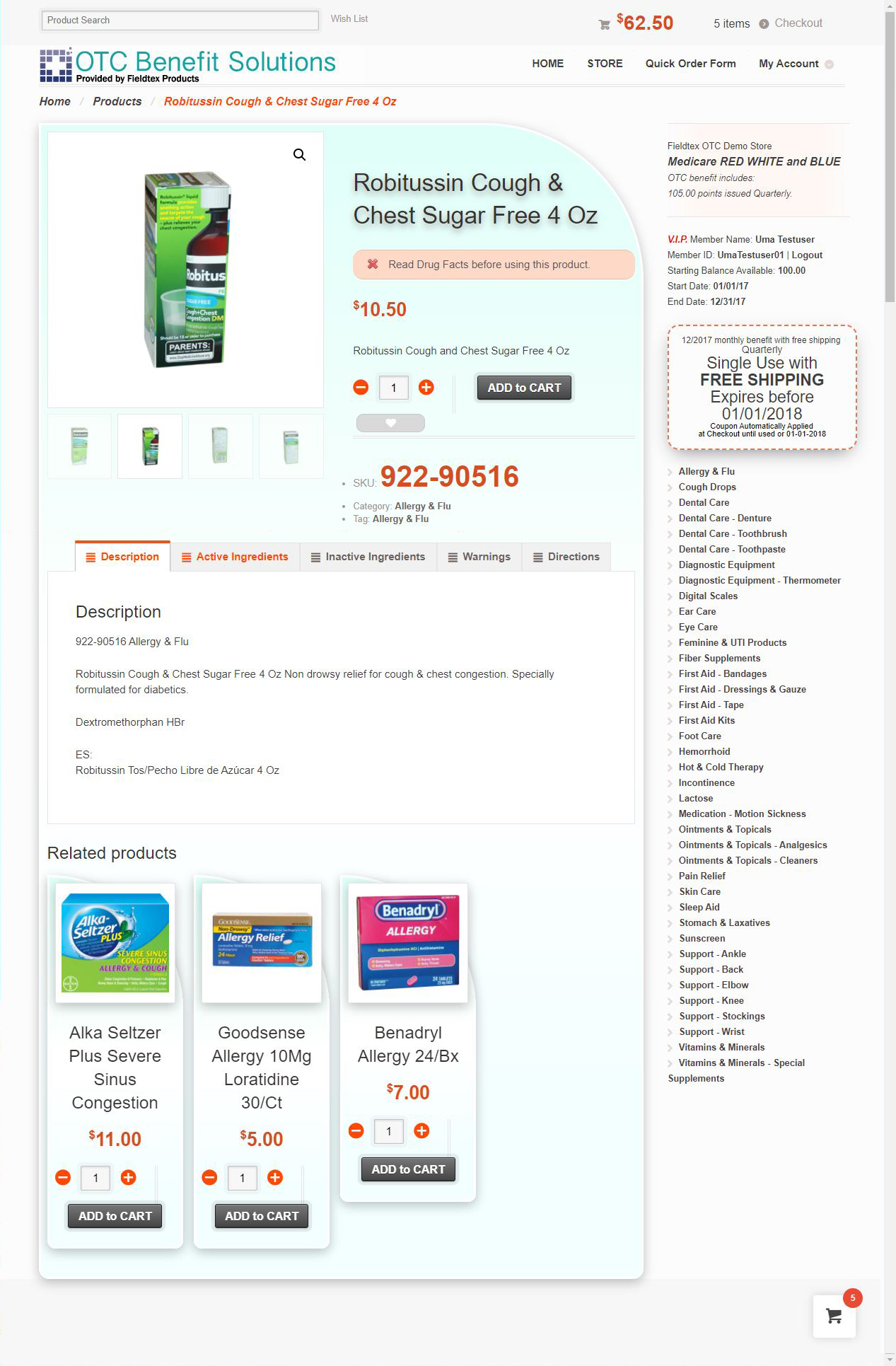This screenshot captures an online product listing from a service titled "OTC Benefit Solutions," provided by FLED Tech Products. Displayed prominently in the center of the screen is an item, Robitussin Cough and Chest Sugar-Free, 4 ounces, packaged in a green box featuring a picture of the product bottle. The product details emphasize the need to "read drug facts before using this product" and indicate the price of $10.50. The display shows an adjustable quantity selector, starting from one unit, along with an "Add to Cart" button. 

Additional noteworthy details include the presence of yellow and navy-colored text on the box, and a SKU number located at the lower section of the screen. The interface also highlights various clickable product categories arranged vertically on the right side, aiding in navigation. Further down, the description of the Robitussin product elaborates on its features and benefits, making it easier for consumers to make an informed purchasing decision.